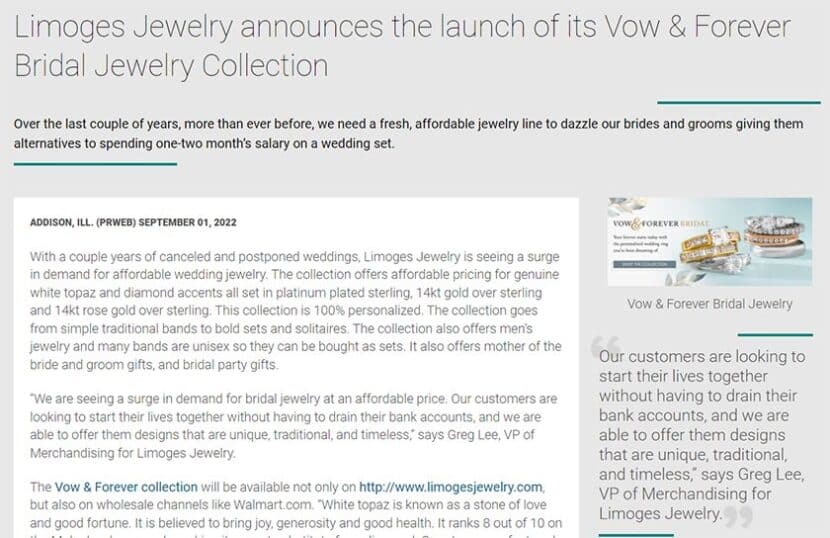**Limoges Jewelry Announces Launch of the Vow and Forever Bridal Jewelry Collection**

This announcement screenshot features a gray background with prominent text at the top stating: "Limoges Jewelry announces the launch of its Vow and Forever Bridal Jewelry Collection." The text elaborates on the collection's goal to provide an elegant, affordable alternative for brides and grooms, allowing them to opt for dazzling jewelry without spending one to two months' salary on wedding sets. 

Dated September 1st, 2022, from Addison, Illinois, via PR Web, the announcement explains how the pandemic has led to a surge in demand for affordable wedding jewelry after numerous canceled and postponed weddings. The collection features genuine white topaz and diamond accents set in platinum-plated sterling, 14-karat gold over sterling silver, and 14-karat rose gold over sterling silver, all at accessible price points. Personalization is a key aspect, offering everything from simple traditional bands to bold sets and solitaires. Men's jewelry and unisex bands suitable for sets, as well as mother-of-the-bride and groom gifts, and bridal party gifts, are also part of the collection.

Greg Lee, VP of Merchandising for Limoges Jewelry, emphasizes that their customers seek to start their lives together without depleting their savings, and the collection meets this need with unique, traditional, and timeless designs. The Vow and Forever Collection will be available on Limoges Jewelry's official website and retail platforms such as Walmart.com. The detailed photograph on the right showcases several diamond rings in gold, silver, and platinum settings, underscoring the charm and variety of the collection.

Underneath the rings, text reiterates Greg Lee's statement: "Our customers are looking to start their lives together without having to drain their bank accounts and we are able to offer them designs that are unique, traditional and timeless." 

Overall, this image powerfully communicates Limoges Jewelry's effort to cater to budget-conscious couples seeking quality and elegance in their bridal jewelry.